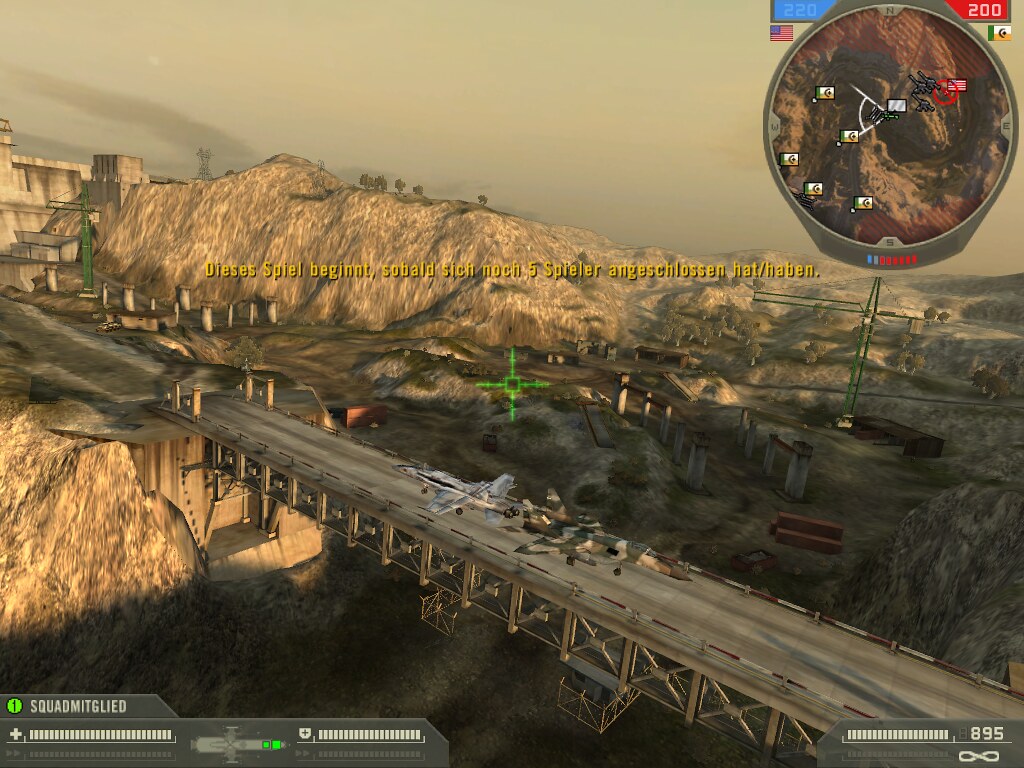The image appears to be a screenshot from a war-themed video game featuring a player flying a jet aircraft. At the bottom of the screen, an infinity symbol is displayed, likely indicating that the player has unlimited ammunition. The player has a stat reading "895," which may represent their current health or the durability of the vehicle.

Text in a foreign language is visible on the screen. It reads, "Dieses Spiel beginnt sobald sich fünf Spieler eigenkannassen haben," which translates from German to "The game begins as soon as five players have chosen their classes." This suggests that the game is likely of German origin.

In addition, there are two flags displayed; one is an American flag, and the other is a green, yellow, and white flag, possibly representing another nation or faction within the game. The term "Squad McGlide" is also present on the screen, though its significance is unclear.